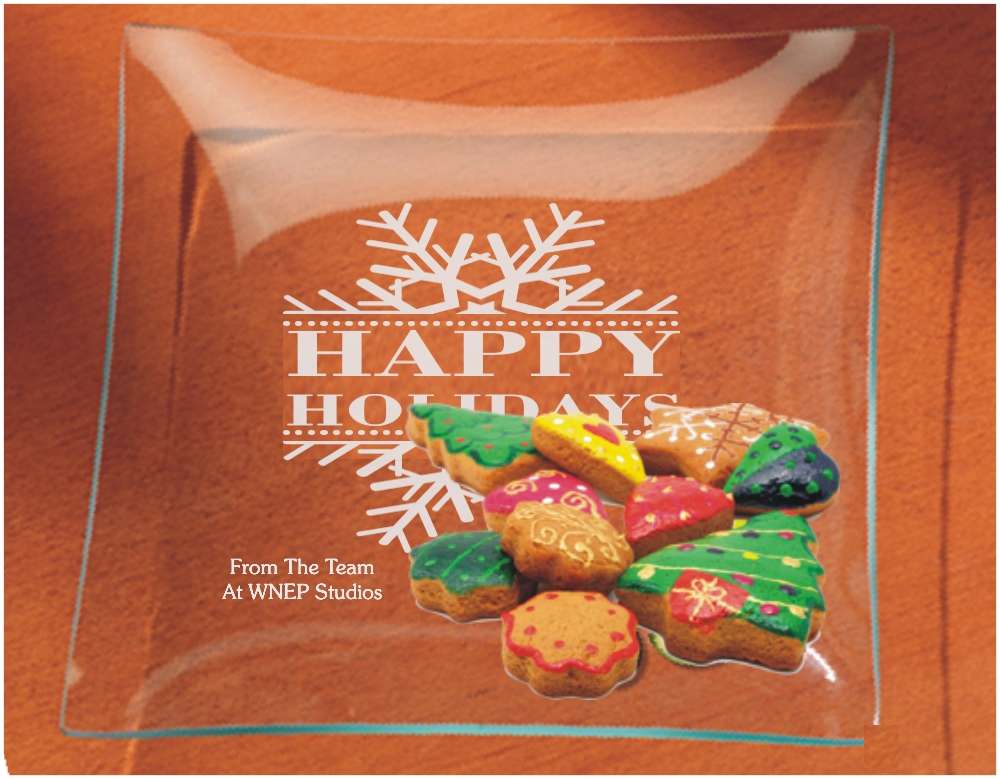In this image, we see a clear glass bowl containing an assortment of decorated Christmas cookies, including tree-shaped cookies with icing ornaments and round cookies. The bowl is placed on a brown wooden table and reflects a distinct orange background. Several reflections and glares on the glass bowl can be observed, adding a touch of vibrancy to the scene. 

Centered on the bottom of the bowl is a white snowflake logo with the text "Happy Holidays" prominently displayed in capital letters, framed by dashed lines above and below, and additional diagonal lines extending from the snowflake. Below the festive message, there's a note that reads "From the Team at WNEP Studios," indicating that this is likely a holiday gift from the studio's team. The image, despite its cheerful content, appears to have been digitally altered, particularly noticeable in the placement of the cookies inside the bowl.